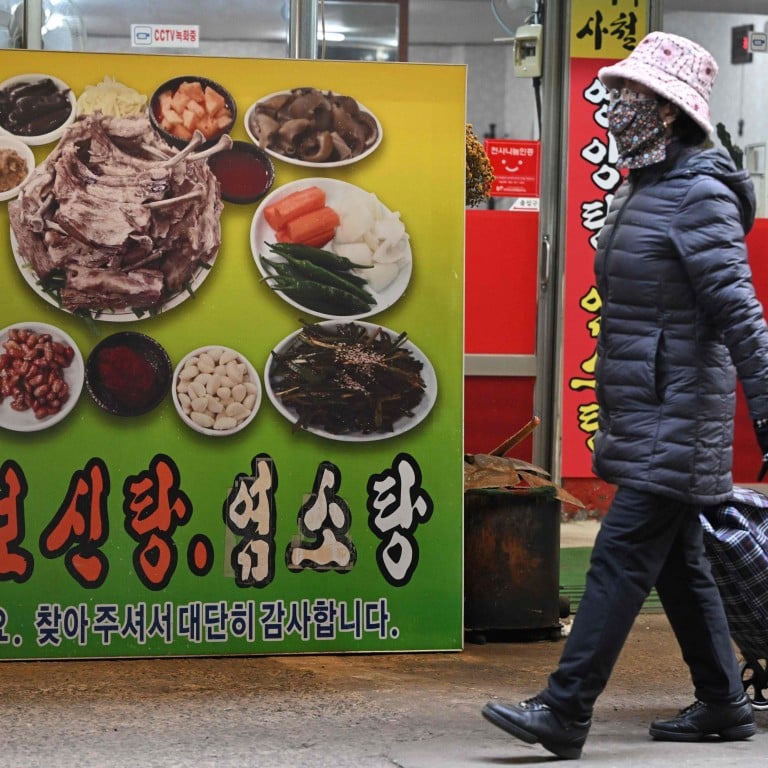In this close-up street scene, a woman, likely a grandmother, is walking on the right side of the frame. She is dressed warmly in a black puffer jacket, black pants, and black shoes, and she sports a decorative cloth face mask along with a light pinkish fishing cap. She is pulling a wheeled valise case that seems suited for carrying groceries. To the left of the image stands a large advertisement poster, approximately five feet by six feet, featuring pictures of various Korean food dishes with Korean text. In the background, the façade of a store with red Korean writing and a door is visible, contributing to the urban setting of this photograph.